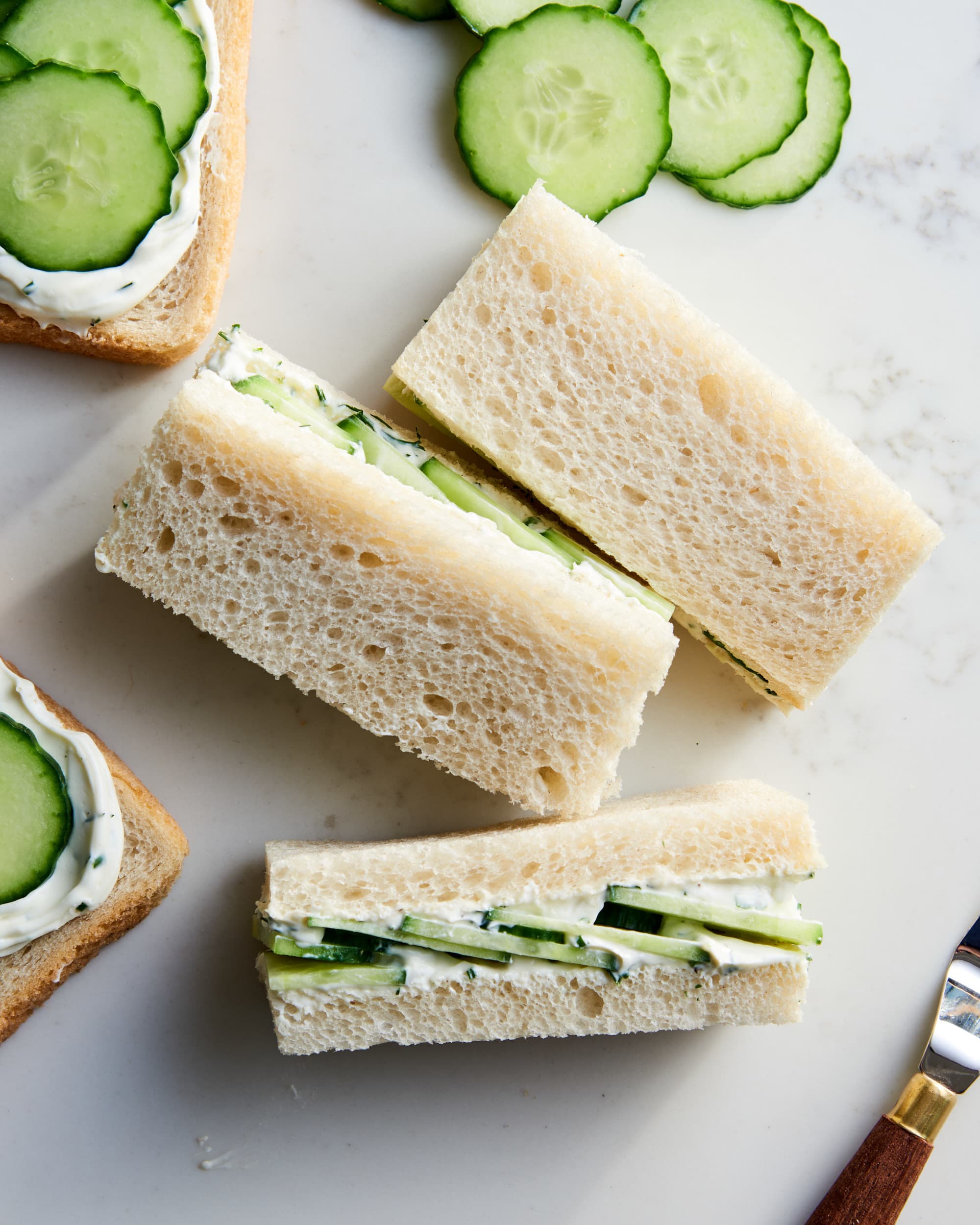The photograph captures a close-up view of a prep station, likely set for a British tea party, featuring an array of cucumber finger sandwiches on a white, marble countertop flecked with shades of gray and black. The centerpiece of the image showcases three neatly arranged finger sandwiches made from crustless white bread. One sandwich lies on its side, revealing a sumptuous layer of cream cheese mixed with herbs like chives or dill, and thin slices of cucumber. Adjacent to the main sandwiches, the upper right portion of the image displays neatly arranged cucumber slices. In the left sections of the image, there are partially assembled sandwiches with crusts still intact, showcasing layers of creamy spread and cucumber awaiting their top bread layer. A serving knife or utensil is casually placed in the bottom right corner, hinting at the ongoing preparation. The overall composition is simple yet elegant, highlighted by the muted colors of white bread and cream cheese, contrasted by the fresh green of the cucumbers, under soft lighting originating from the upper right.